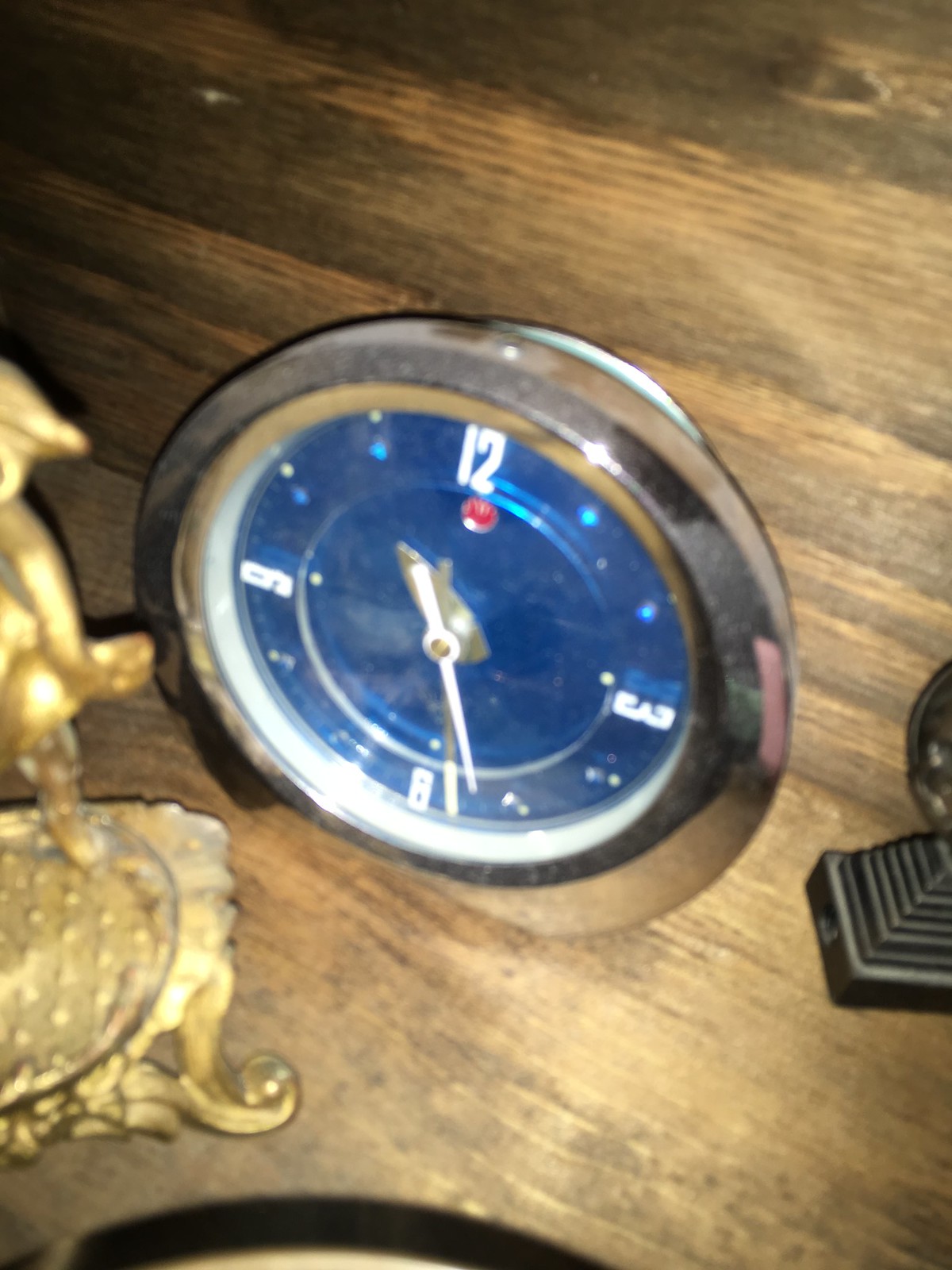This detailed photograph showcases a small, inset clock within a medium-colored, distressed wooden piece. The clock features a vivid navy blue face surrounded by a metallic silver ring. Only the numbers 12, 3, 6, and 9 are marked in white with blocky font, while the other hours are represented by bright blue dots. The clock's minute hand is in white and the hour hand is brass-colored. The hands are positioned at approximately 6:30. Below the 12, there is a red dot. To the left of the clock, there is a gold-colored ornamental sculpture, partially visible, resembling a shell with wavy lines, though it is mostly off-camera. On the far right, a portion of a dark-colored pyramid-shaped pedestal with a round object on top can be seen, also mostly off the edge of the image.